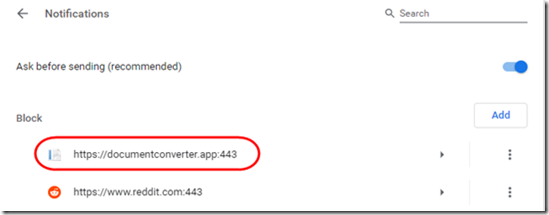The image depicts a user interface with a clean, white background, bordered in black on the right side. In the top left corner, an arrow labeled "Notifications" points to the left. On the top right, a magnifying glass icon labeled "Search" is present. Just below these elements, a horizontal line spans the width of the interface, providing separation.

Further down on the left side, there is a text label that reads "Ask before sending (recommended)" with a blue toggle switch to the right that is in the "on" position. Below this, another label on the left reads "Block," accompanied by an "Add" button on the right.

Underneath the "Block" section, there are two URLs listed:

1. "https://documentconverter.app:443" circled in red.
2. "https://www.reddit.com:443"

To the right of each URL, there is a vertical ellipsis, indicating additional options are available.